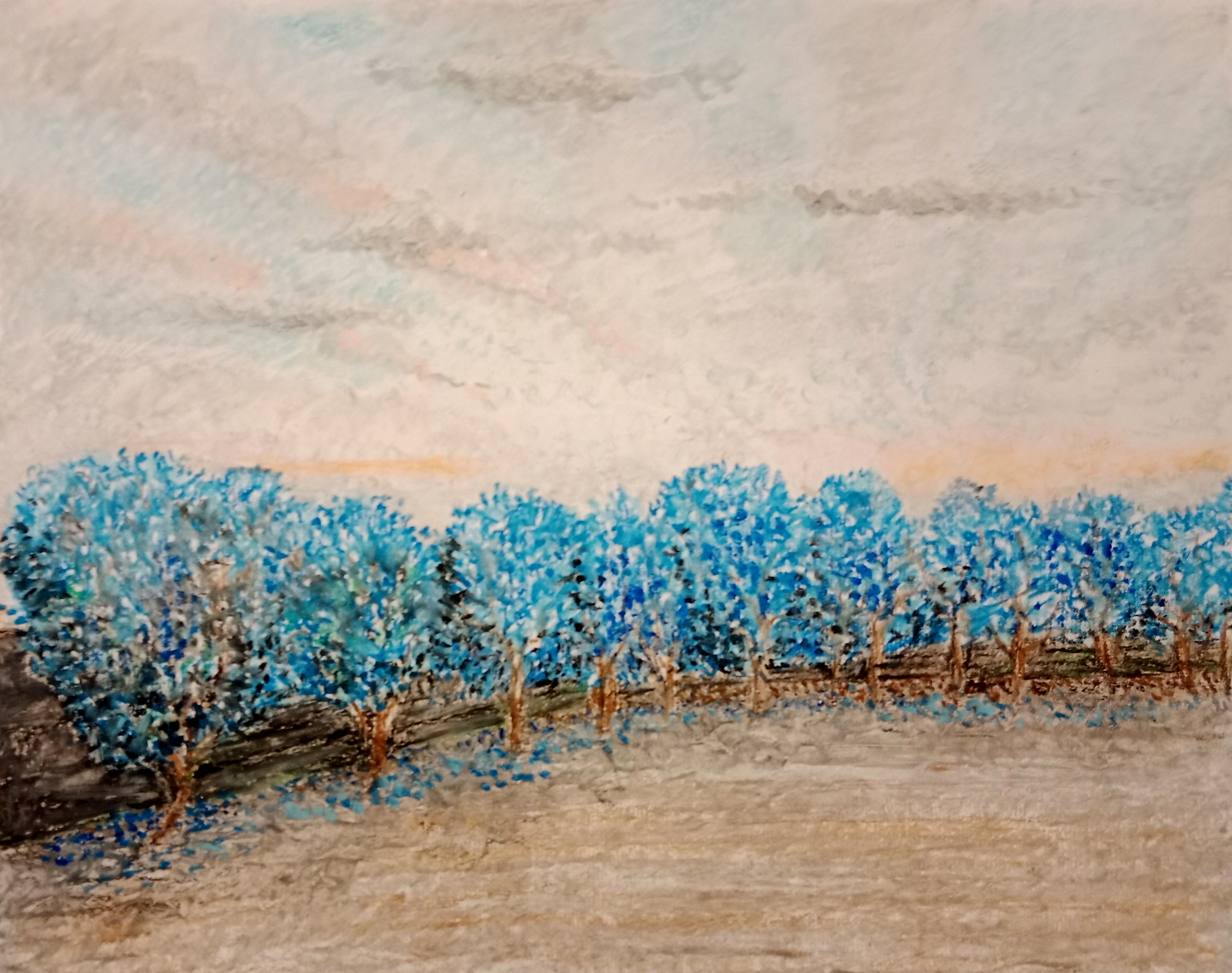This color image, possibly a line drawing or a painting, showcases a serene landscape predominately rendered in soft pastels with intricate pencil details. The foreground features a textured ground area composed of varying shades of brown and grey, meticulously filled in with lighter and darker tones. A line of trees spans the entire width of the image, their round forms blending into one another, creating a nearly continuous canopy. These trees, featuring brown trunks, are adorned with blue leaves, with one tree second from the right, uniquely bearing some green foliage. Despite their merging outlines, at least ten trees are discernible, adding to the composition's depth.

Above this tranquil scene, a pastel-hued sky unfolds. The lower portion of the sky is dominated by a cream tone, accented with thin, horizontal orange clouds. Ascending upwards, a subtle sunray effect emerges, characterized by delicate rays of very pale orange or brown. The sky further features patches of bluey-green, harmoniously blended into the pastel scheme. Enhancing this atmospheric effect, thin horizontal grey clouds are lightly penciled in, adding a muted, ethereal quality to the overall composition.